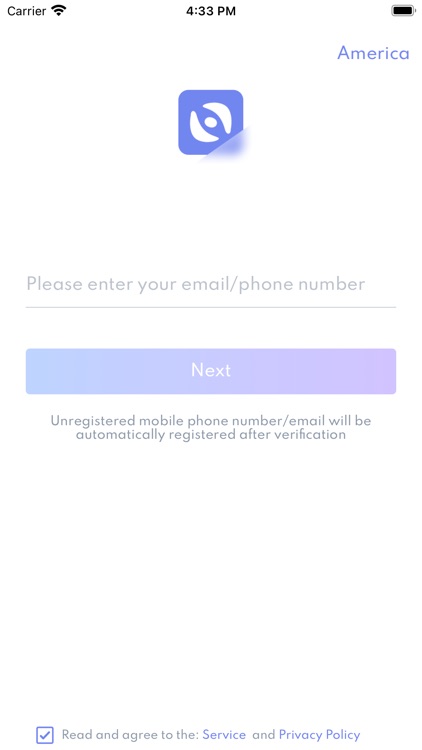This is a detailed screenshot of a smartphone's screen captured in a vertical orientation, prominently displayed in the upper left-hand corner. At the very top of the screen, the word "Carrier" is visible, indicating the network provider. To the right of "Carrier," a Wi-Fi signal icon is present. Centrally placed at the top, the time is displayed as "4:33 PM." In the upper right-hand corner, the battery icon shows a full charge.

Directly below the battery icon, the word "America" is written in purple text. Moving to the top center of the screen, a square logo with rounded corners is visible. This logo is purple, featuring a circular design in the middle, encircled by two broad, curved lines.

In the center of the screen, text prompts the user to "Please enter your email / phone number." Just below this prompt, there is a "Next" button, styled in purple with white text. Further down, a message states, "Unregistered mobile phone number / email will be automatically registered after verification."

At the bottom of the screen, there is a notice requesting the user to "read and agree to the service and privacy policy."